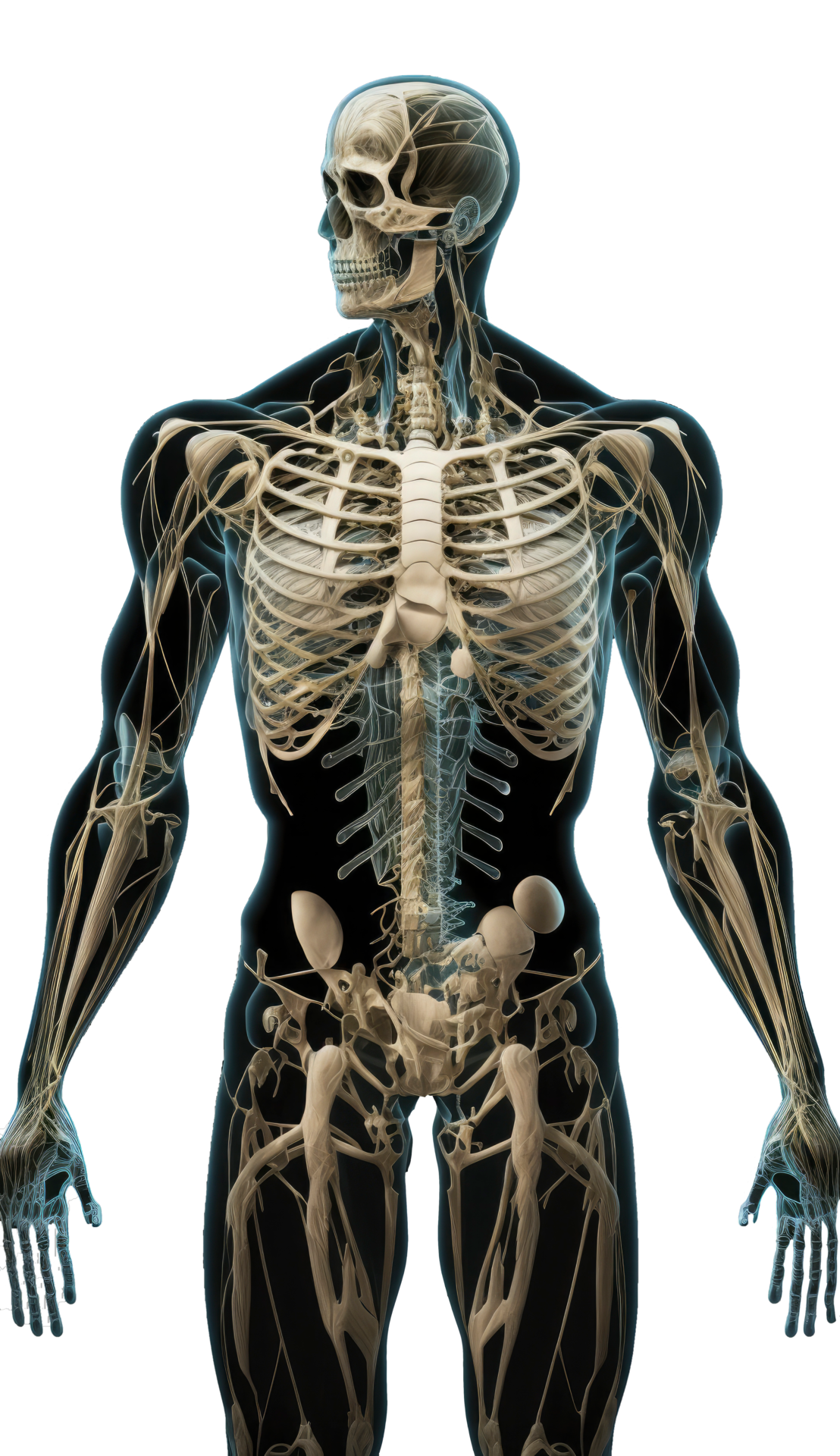This detailed anatomical illustration features a black silhouetted figure of a muscular man against a pure white background, displayed from head to knees with the head turned to the left. Overlaid on the silhouette is an intricate x-ray style depiction of the human skeletal structure in various hues, primarily beige with shades of blue accentuating certain areas such as parts of the fingers, hand, and specific nerve pathways around the neck and down the spine. This comprehensive imagery also reveals stringy objects resembling ligaments or veins in a beige color similar to the bones. The skull exhibits a smooth muscle-like pattern at the back of the face. The entire depiction presents a detailed and layered view of the underlying bones, muscles, nerves, and ligaments, offering an in-depth look at the internal composition of the human body.